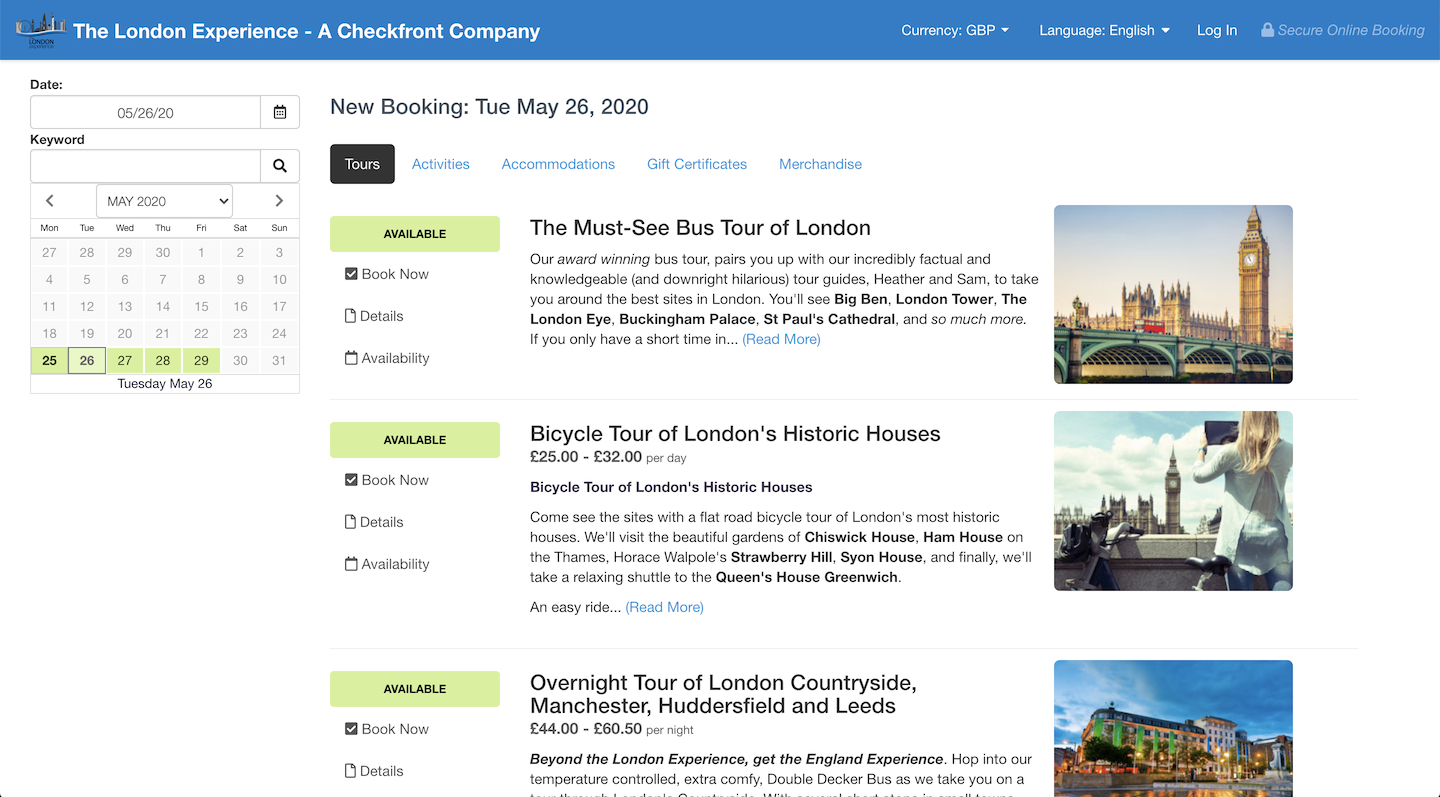This image showcases an online booking website titled "The London Experience, Czech Front Company," prominently displayed in the top left-hand corner. The white background creates a clean and organized look. In the bottom right-hand corner, three photographs of various iconic London buildings suggest the site's primary focus on London tourism.

On the left side of the page, a list of various articles and titles describes different London destinations, along with the average price range for visiting each site, indicating the website's function as a booking platform. The interface appears set for a travel period of a full week, specifically from Tuesday, May 26, 2020.

In the top right-hand corner, there are buttons for user login, language selection, and currency adjustment. The current settings show English as the selected language and GBP (British Pounds) as the chosen currency. Additionally, a calendar icon located in the top left-hand corner highlights the month of May, with five dates—May 25th to 29th—marked in light green, signaling potential booking dates.